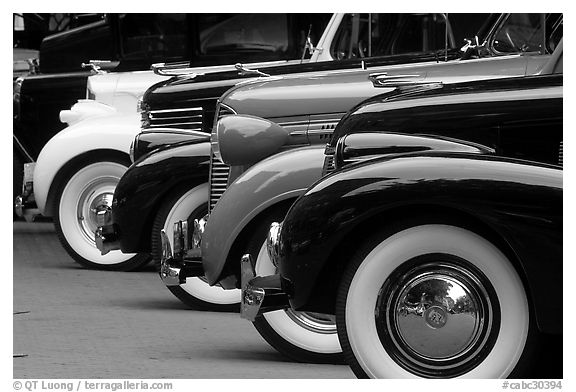The black and white photograph showcases a lineup of five classic cars from the 1920s or 1930s, prominently displaying the cars' front wheels and hoods. Three of the cars have dark colors, one is a moderately dark shade, and one is white. Each car features distinctive hood ornaments and white-rimmed tires, exuding a sporty and elite aesthetic. While no drivers are present, the cars stand out in their timeless elegance. At the bottom of the image, a credit reads "Photo by Katie Luong from TerraGalleria.com".